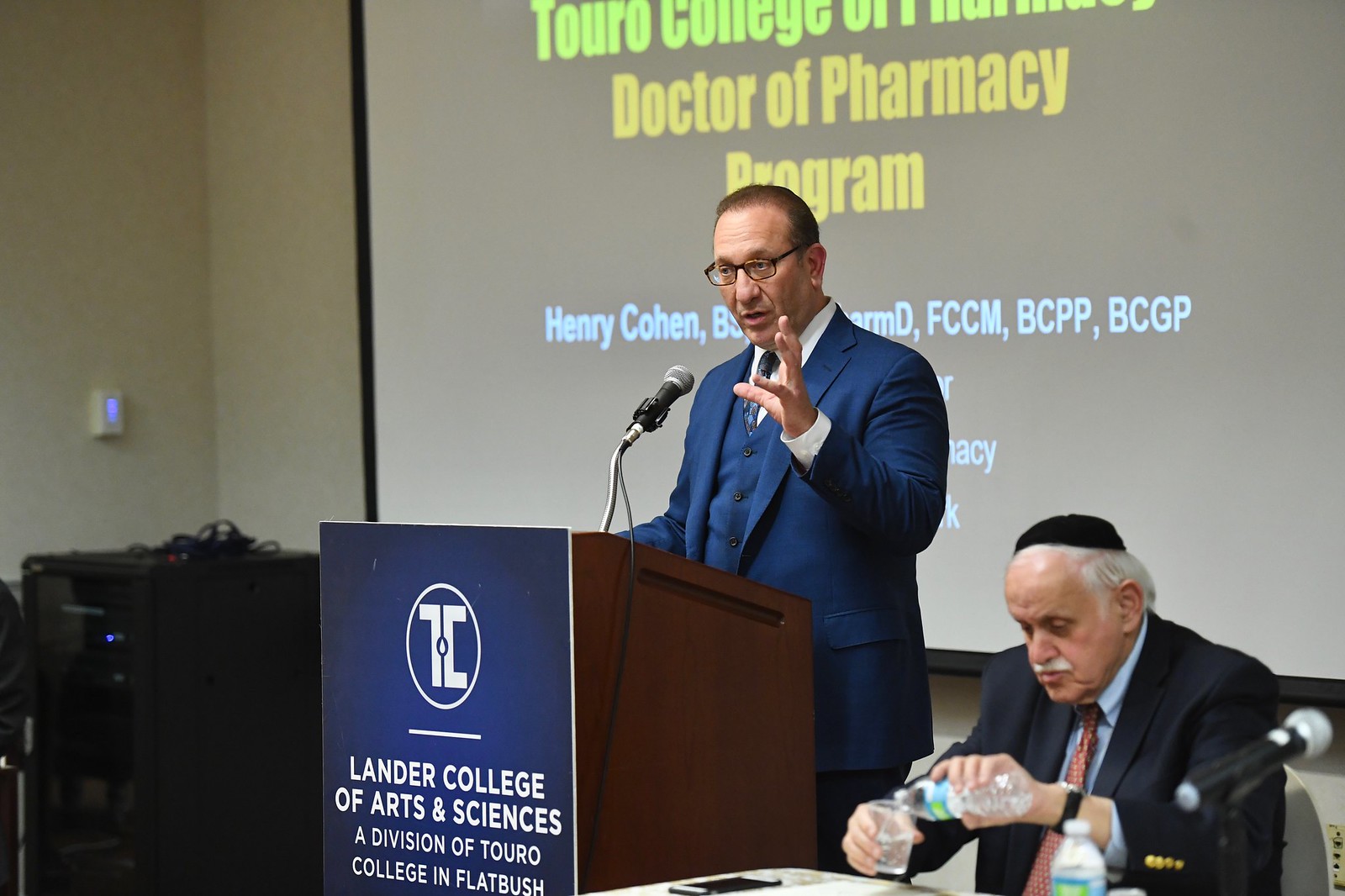This detailed, color photograph captures an indoor event featuring two men in dark blue suits. The focal point is a man standing at a podium, labeled with a sign that reads "Lander College of Arts and Sciences, a division of Touro College in Flatbush." He is speaking into a microphone with one hand raised. Behind him, a white projection screen displays the words "Doctor of Pharmacy Program" and the name "Henry Cohen," along with a list of achievements partially obscured by the speaker's stance.

In the foreground, an older gentleman with gray hair and a mustache, wearing a yarmulke, is seated. He is pouring water from a bottle into a glass. This man also has a microphone nearby, and an iPhone is visible on the table in front of him. The scene appears well-organized, suggesting an academic or professional setting focused on the Doctor of Pharmacy program.